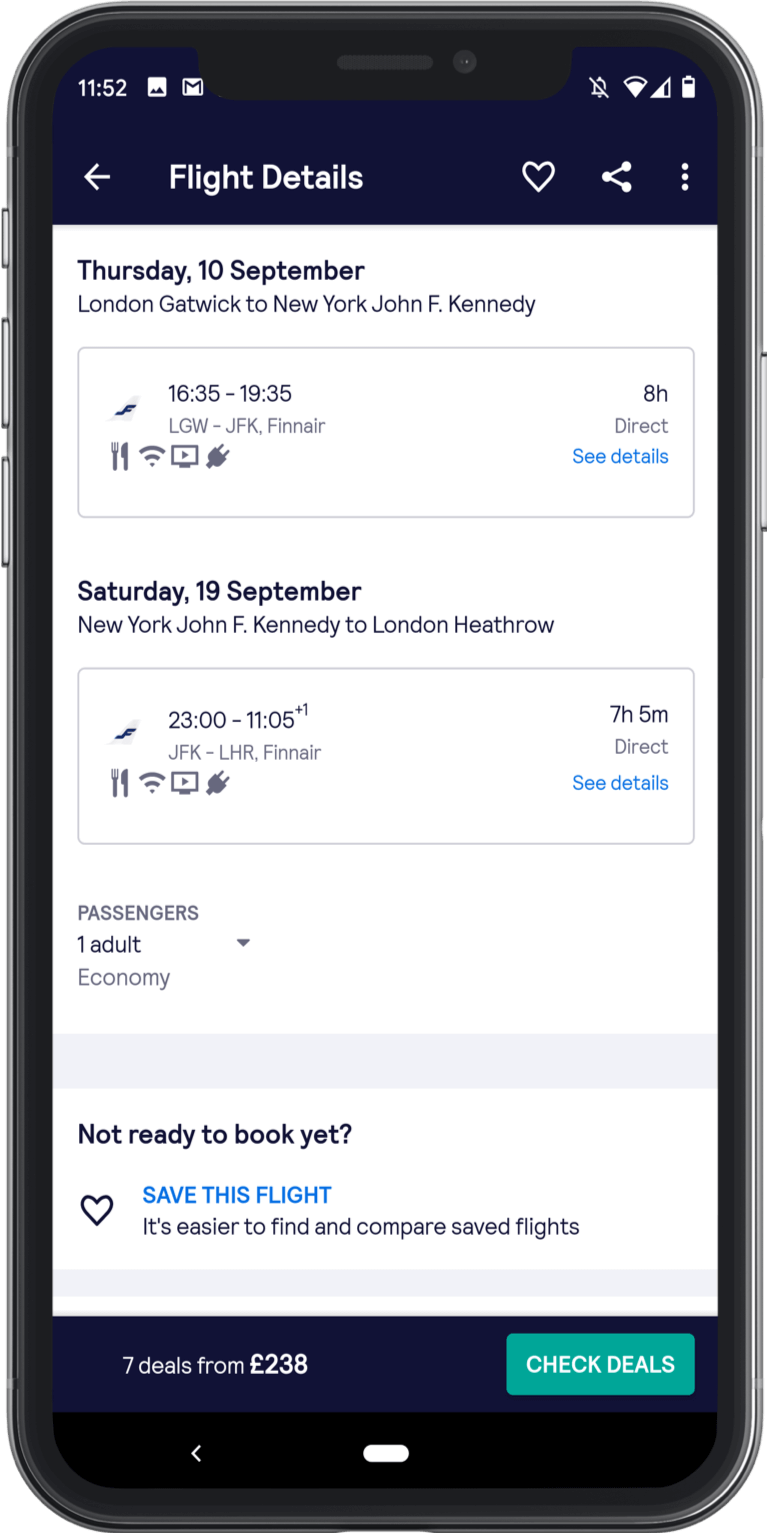A detailed mock-up of a smartphone display is showcased, bordered by a sleek black bezel. The clock on the top left reads 1152, suggesting military time due to the absence of AM or PM designations. Adjacent to the clock is an image placeholder icon—a white square featuring a black mountain design. The screen includes common app icons such as Google and Gmail.

On the top right, a bell icon with a diagonal line through it signals some notifications are muted. Next to it, icons for a strong Wi-Fi connection, full cellular signal, and a nearly full battery are visible. A bold white arrow points towards the text "Flight Details," flanked by interactive icons including a heart, a share symbol, and three ellipses.

The primary text area displayed is a detailed itinerary for a round trip between London Gatwick and New York John F. Kennedy. Bold black text announces, "Tuesday, 10 September," followed by thinner text detailing the flight route: "London Gatwick to New York John F. Kennedy." Departure and arrival times are 1635 and 1935, respectively. The flight, coded LGW - JFK, is operated by Finnair and offers onboard amenities such as food, Wi-Fi, television, and charging outlets. The direct flight duration is 8 hours, with a hyperlink for additional details.

Following this, a return flight is highlighted for "Saturday, 19 September," from New York John F. Kennedy to London Heathrow. Departure is at 2300 and arrival is at 1105 the next day. This leg of the journey, coded JFK - LHR, also operated by Finnair, includes the same onboard services and has a flight duration of 7 hours and 5 minutes. 

A bottom section specifies passenger details: "One Adult" with a dropdown menu option, and the travel class is marked as "Economy." A call-to-action rectangle states, "Not ready to book yet?" in bold text, followed by an invitation to "Save this flight," in bold blue text, indicating it’s easier to find and compare saved flights thereafter.

The bottom portion features a dark blue rectangle with the text, "7 deals from," followed by "£238" in bold white. A teal button labeled "Check Deals" appears to the right. The phone's bottom bezel includes a left-pointing arrow for navigation and an oval button at the center, presumably for multitasking or screen navigation.